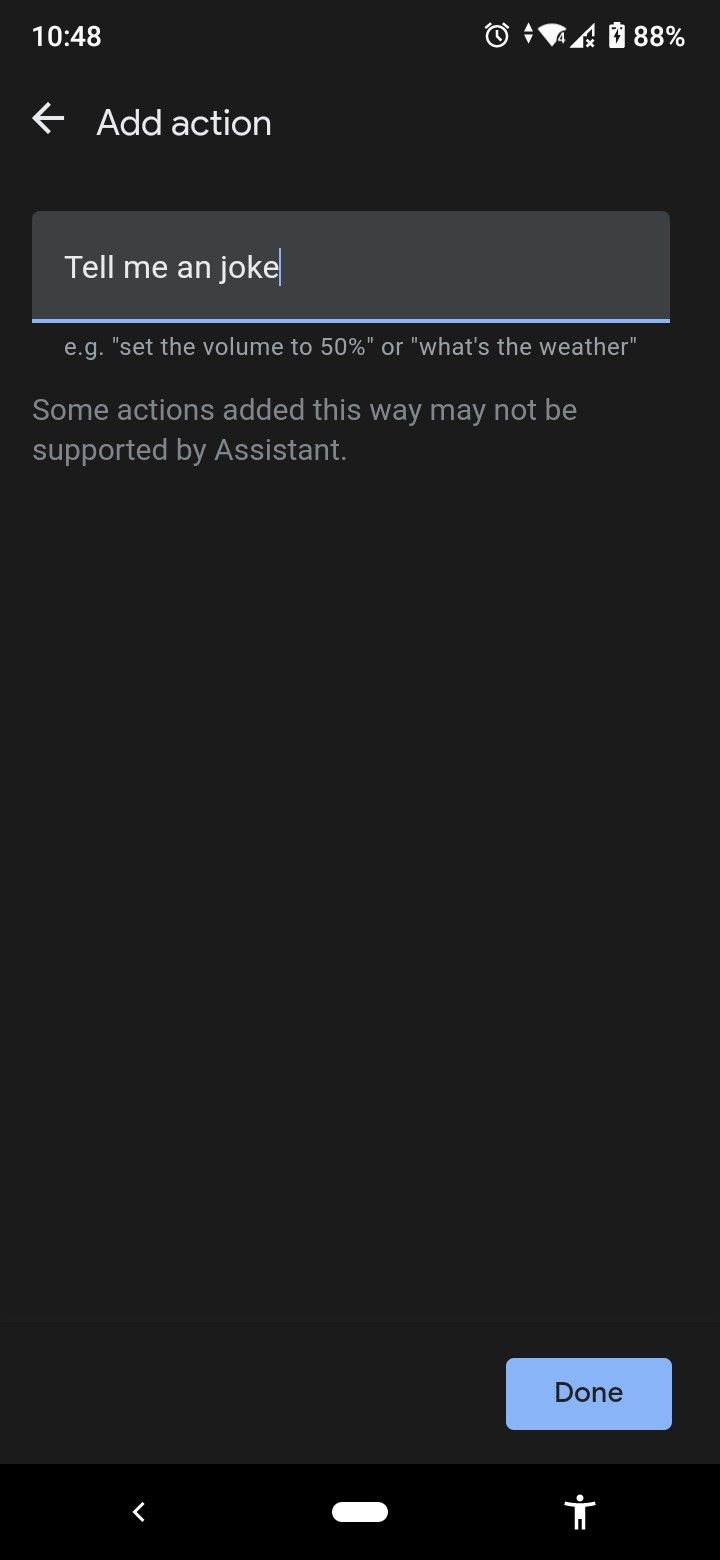In this detailed screenshot of a smartphone interface, the status bar at the top reveals a time of 10:48 and a battery level at 88%, with the phone currently charging. Beneath the status bar, there's an interface featuring an "Add Action" label near the top left and a back button to its immediate left. The central portion of the image showcases a text input box containing the words "tell me a joke," with placeholder text below the box suggesting commands like "set the volume to 50%" or "what's the weather." A subtitle warns that some actions added through this interface may not be supported by the Assistant. The rest of the section features a dark gray background. In the bottom right corner, there is a blue rectangle with the word "Done" in black text. At the bottom edge of the screen, typical navigation buttons appear: a back arrow, a home button, and a small person icon representing a profile or accessibility option.